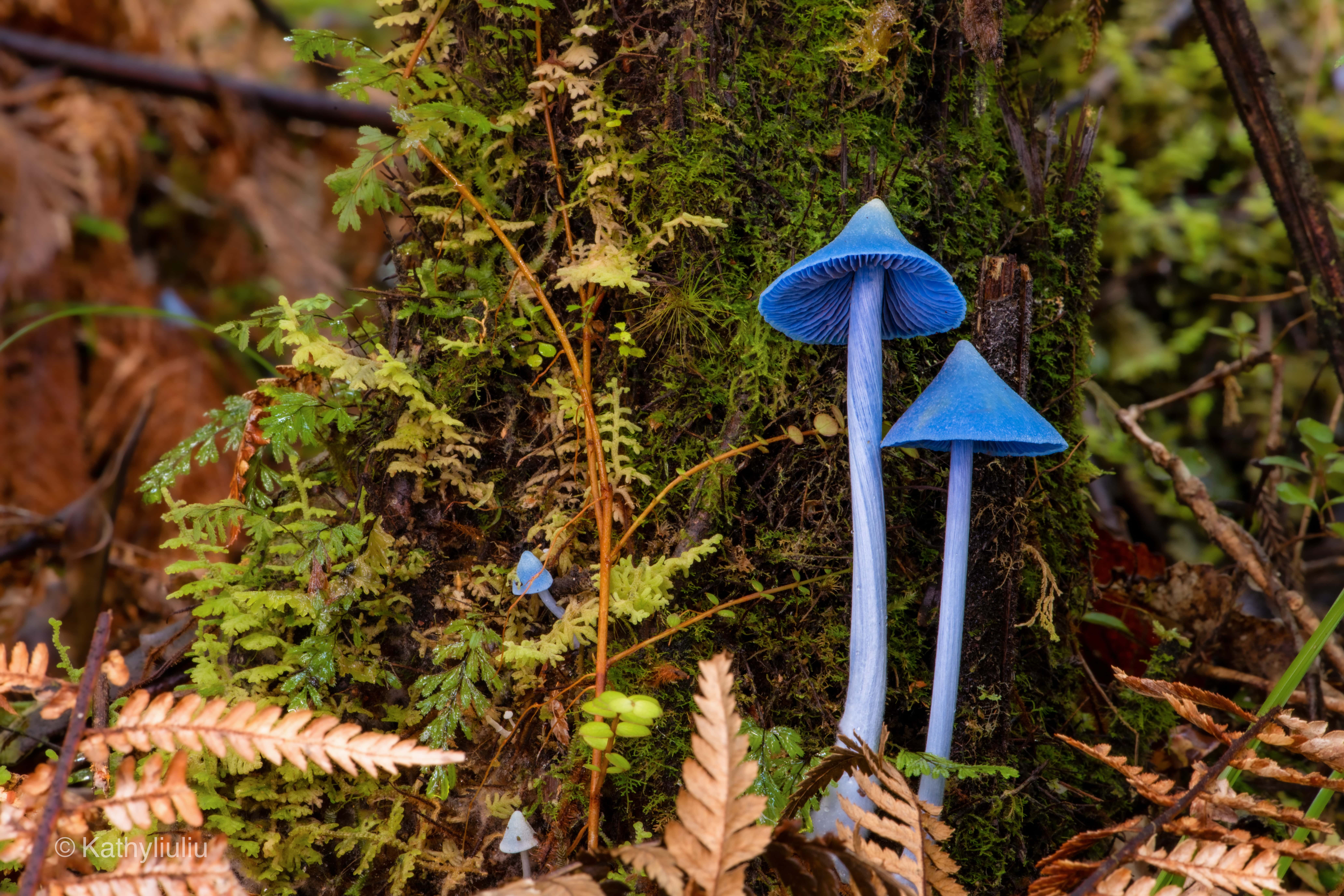In this captivating image by Kathy Liuliu, we are immersed in a dense, forested setting dominated by a large tree with its trunk gracefully covered in moss. The scene showcases a pair of strikingly beautiful blue mushrooms with tall, slightly bluish-white stalks and conical caps that transition to a hint of white at their peaks. These mushrooms, two larger and two smaller ones, serve as a focal point against the lush background of green ferns, brown leaves, and other forest flora, with some vegetation appearing wilted and brown. The overall palette of the photograph features vibrant greens and browns, with the bright blue mushrooms bringing a pop of color and a sense of magic to the composition. The atmosphere appears to be overcast, with diffused lighting that lends a serene and somewhat mystical quality to the scene. Notably, the image carries a watermark at the bottom left, indicating the photographer's name, Kathy Liuliu. This beautifully detailed and enchanting nature shot vividly captures the essence of a northern hemisphere forest.